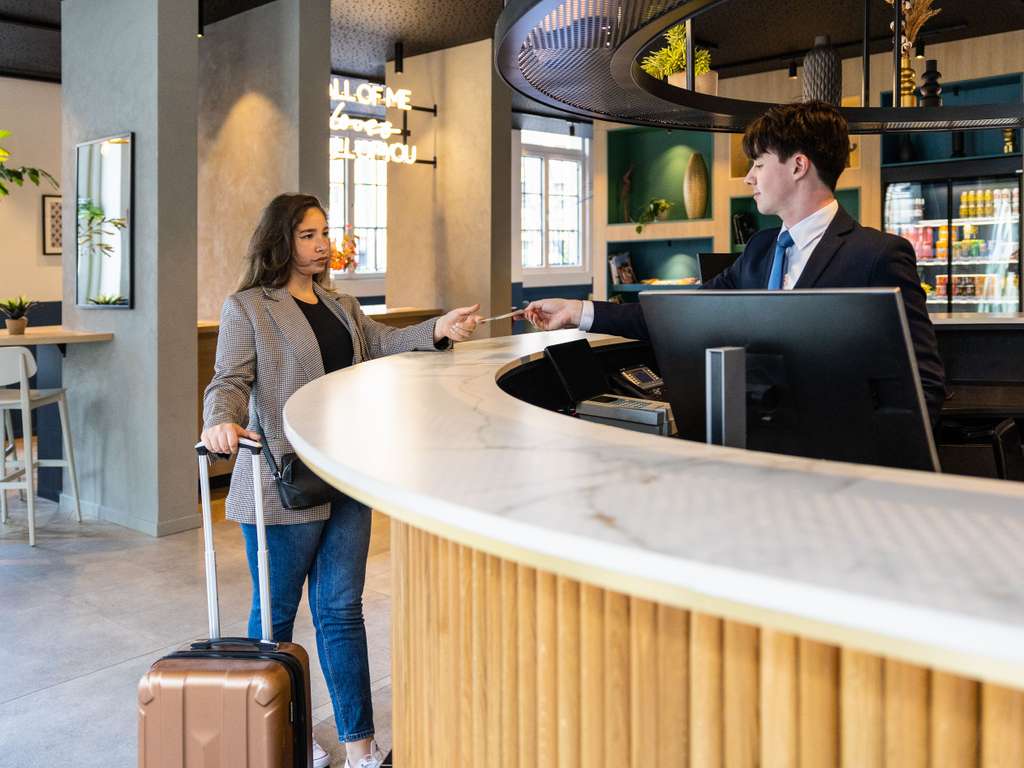The image depicts a modern reception area, possibly a hotel lobby or a coffee shop, with a white curved counter fronted by bamboo-style paneling. A woman stands at the counter, wearing a light gray menswear-style jacket over a black top, paired with blue jeans. She has black hair and is carrying a black purse around her waist. Her left hand grips the extended handle of a copper rolling suitcase, while her right hand reaches out to take a ticket or receipt from a young Caucasian man behind the counter. The man, dressed in a black suit jacket, blue tie, and white shirt, stands in front of a black flat panel computer monitor, facing the woman in profile. Behind him, there's a refrigerated case containing various beverages. The background features large windows, light wooden tables with light green-backed chairs, and the floor is covered in gray linoleum. A neon sign in the window reads "all of me," though the remaining text is unclear. The photo is in landscape orientation and captures a sleek, modern aesthetic with great attention to detail.